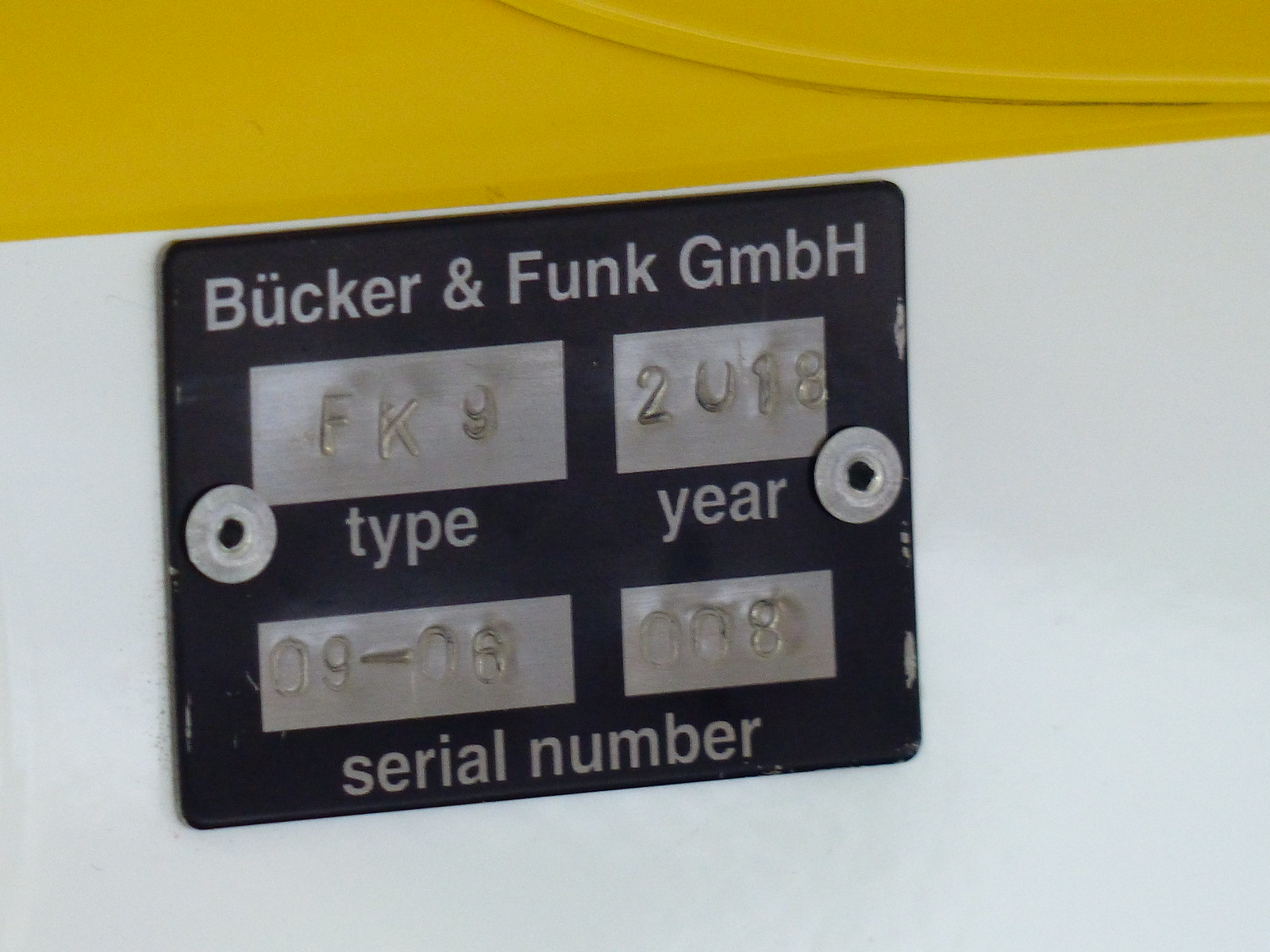The image shows a close-up of a metal identification plaque fastened onto a surface. The mounting surface is white at the bottom and yellow above. The plaque itself is a dark color, possibly black or dark blue, with silver engravings. At the top of the plaque, it reads “Bücker and Funk GmbH.” Below this are four gray rectangles with various inscriptions. The top left rectangle reads “Type: FK9,” while the top right one reads “Year: 2018.” The bottom left rectangle shows a serial number formatted as “0906-008.” This plaque, which appears to be securely riveted into place, likely serves as an identification tag for a piece of equipment or machinery.